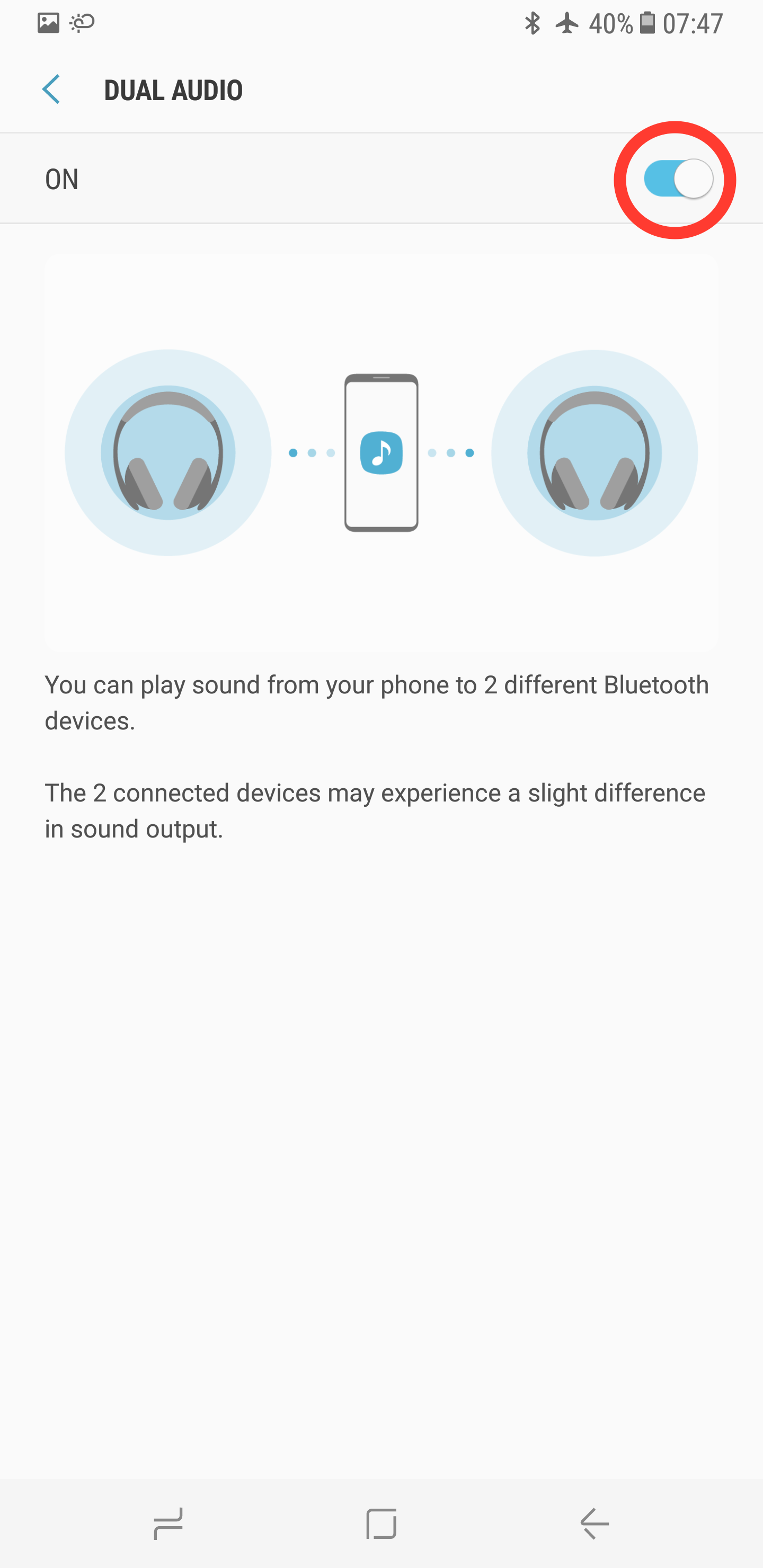Smartphone Interface Showing Dual Audio Settings

The image shows a smartphone interface set against a gray background. The status bar at the top displays a battery level at 40%, the current time as 7:47, a Bluetooth icon, and an airplane mode icon. Below the status bar, the screen highlights the "Dual Audio" feature.

In the center of the display, there is a left arrow symbol and text indicating that the Dual Audio feature is turned on. This is emphasized with a red circle around the toggle bar, which is in the 'On' position. An icon of headphones accompanies this section.

To the left of a phone icon, there is a blue circle containing a music symbol, suggesting music playback functionality. To the right of the phone icon, another headphones icon is present. The description explains that you can play sound from your phone to two different Bluetooth devices, though the two connected devices may experience a slight variance in sound output.

At the bottom of the screen, a gray bar is visible. It resembles an 'L' turned 90 degrees to the left, with another 'L' placed below it. This bar likely represents navigation or an additional interface element.